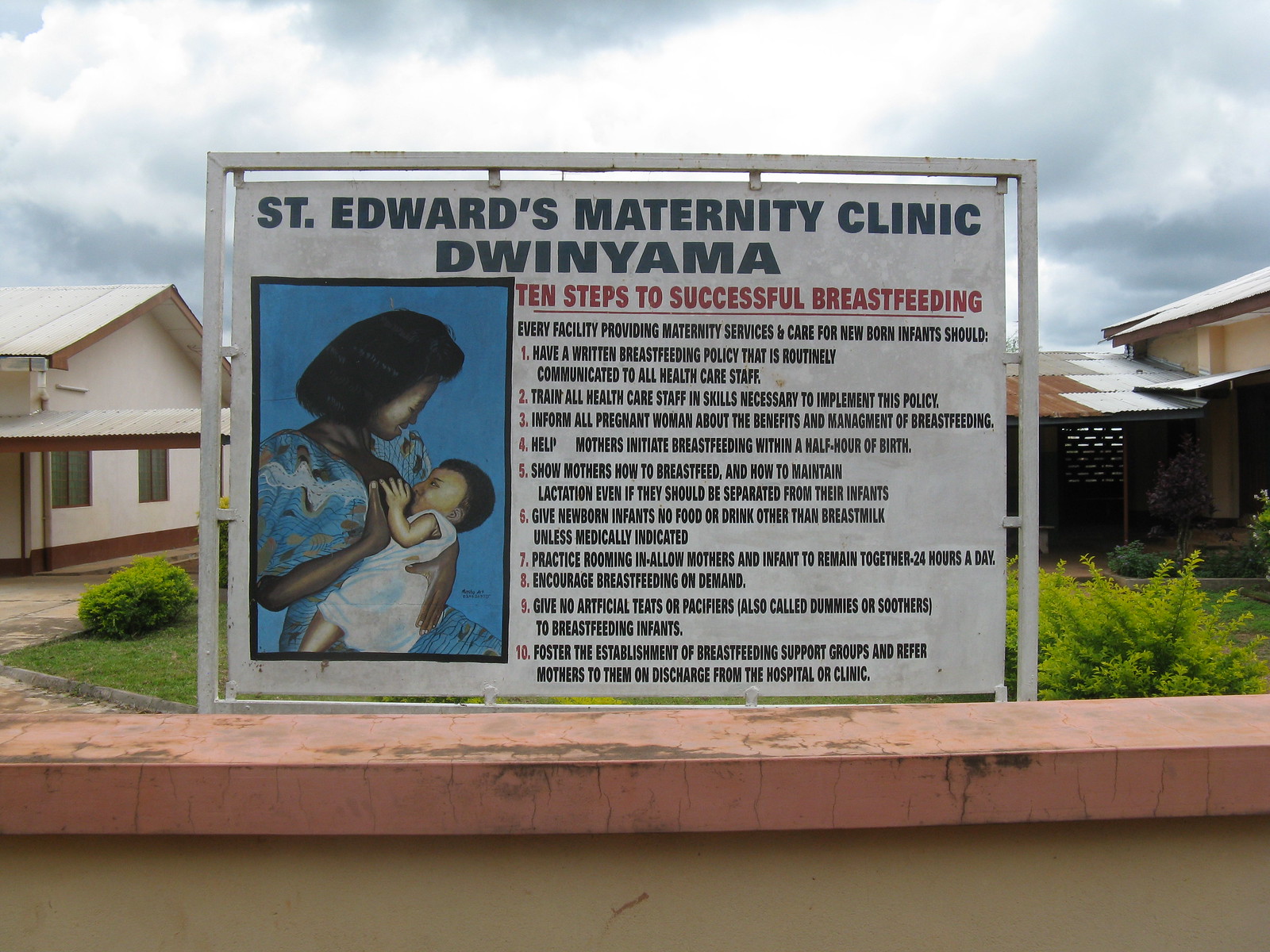The outdoor, daytime photograph captures a detailed scene dominated by a central sign mounted on a pink and cream-colored, worn rail. The sign, framed by a backdrop of brown gabled-roof houses, green plants, and a lawn, heralds "St. Edward's Maternity Clinic DWINYAMA 10 Steps to Successful Breastfeeding." It features an image of a young Asian woman in a blue dress breastfeeding a baby clad in white. The text, written in black, itemizes ten essential breastfeeding principles, urging facilities to adopt policies supporting breastfeeding from birth, educate healthcare staff, and promote continuous mother-infant bonding. The scene integrates a mix of colors—white, gray, blue, black, red, yellow, and pink—against a sky filled with grey clouds, further accentuating the setting's rich details.